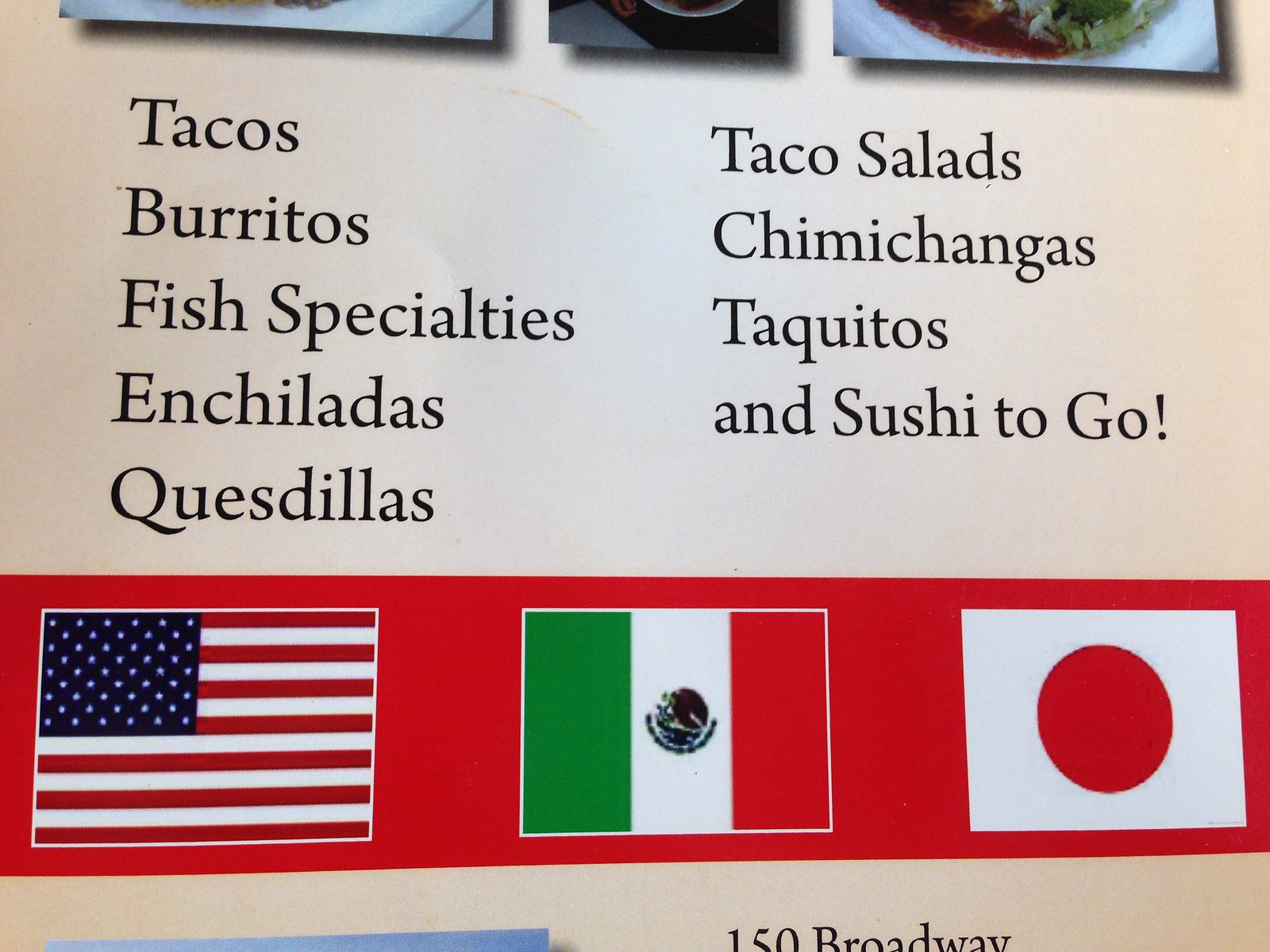The image depicts a wall adorned with a menu showcasing various food items for sale. At the top of the wall, partially visible, are three photographs with the bottoms hanging down, each against a gray backdrop. 

The photograph on the right shows the bottom of a plate containing what appears to be a dish with red sauce. The middle photograph is slightly darker, revealing the edge of a brown plate nested within a white plate, set against a dark gray background.

Beneath the photographs, the menu is divided into two columns. The left column lists "Tacos," "Burritos," "Fish Specialties," "Enchiladas," and "Quesadillas." The right column features "Taco Salads," "Chimichangas," "Taquitos," and "Sushi To Go." 

At the bottom of the menu is a long red rectangle, displaying an American flag, a Mexican flag, and a Japanese flag, each evenly spaced apart. Below this rectangle, though partially cut off by the edge of the picture, the text "122 Broadway" is visible in black.

On the left edge of the bottom part of the wall, the top trim of a piece of paper can be seen, transitioning from light blue to darker blue as it moves leftward. On the wall between the sections labeled "Tacos" and "Taco Salads," there is an orange stain shaped like an arch. The majority of the wall is a light cream color.